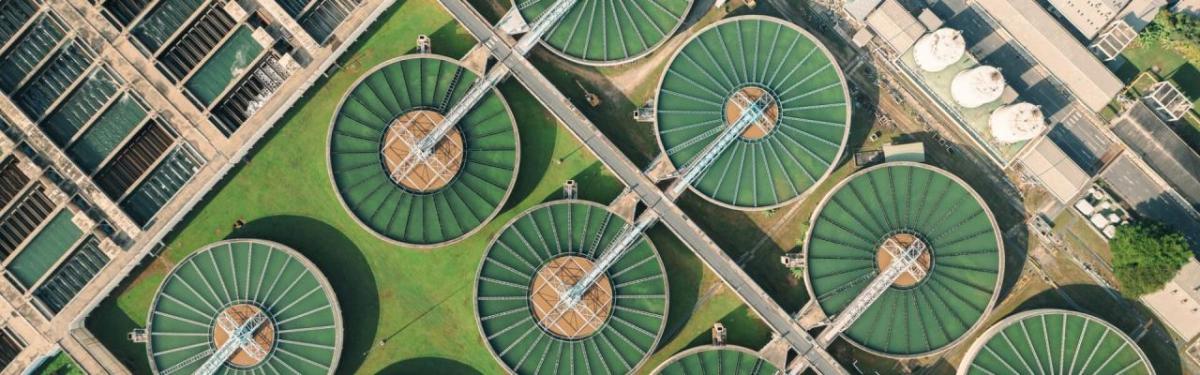The image presents an aerial shot of a vast industrial complex, possibly a refinery or an agricultural storage facility. The photo reveals a series of large, green cylindrical tanks organized in neat rows. Four of these tanks are prominently visible in the mid-right section, while another four can be inferred based on their arrangement. Each tank appears to be interconnected through a network of piping or scaffolding, suggesting the transfer of liquids or gases, and there is a diagonal passageway running between the rows.

Surrounding the primary tanks, additional industrial equipment and storage containers are visible. On the upper right-hand side, there are several rectangular storage vats, further indicating the scale and industrial nature of the site. The complex also includes large rectangular buildings and a prominent cylindrical white container. A thoroughfare or street can be seen bisecting the area, enhancing the impression of an organized and functional facility.

This image, taken from an altitude of approximately 100 to 200 feet, captures the extensive layout and interconnectedness of the site, emphasizing its industrial purpose without providing specific details that clarify its exact function.